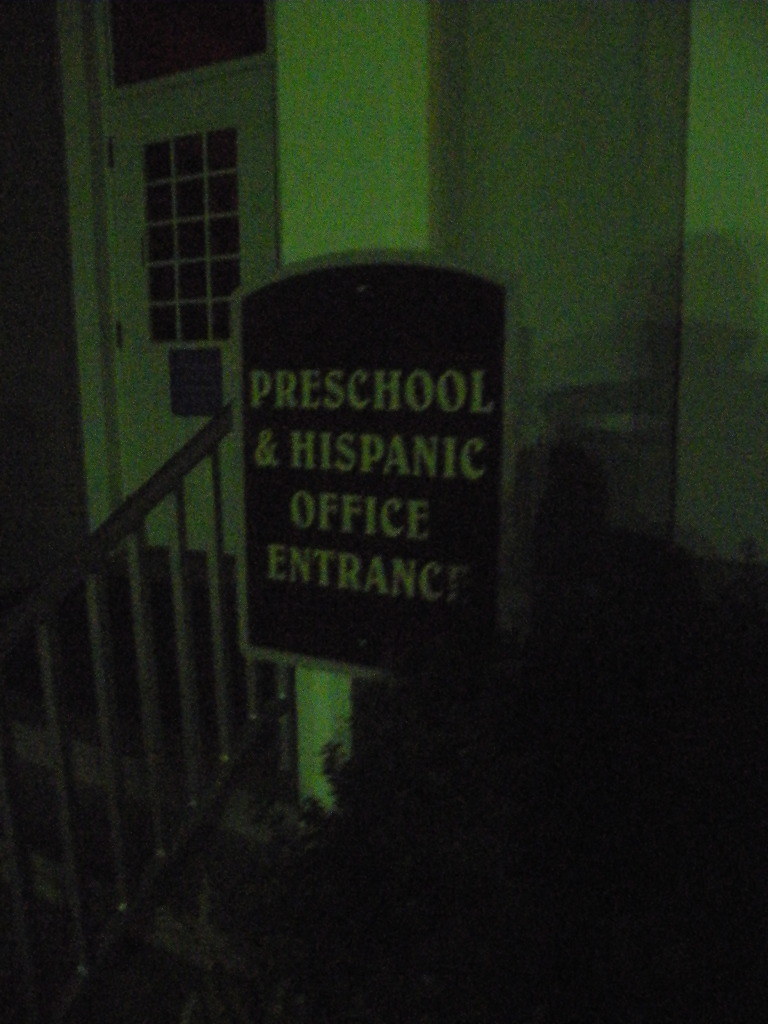The photograph captures a night-time, slightly blurry and dark close-up of a sign mounted on a thick, square pillar. The sign features a gray-brown border with a black center, displaying white text that reads, "Preschool Hispanic Office Entrance." To the left of the sign, a dark black railing is visible, followed by the edges of concrete steps below. The bottom right of the image fades into darkness. In the upper left corner, there is a white-framed door with a small paned window at the top and a black square panel beneath it.